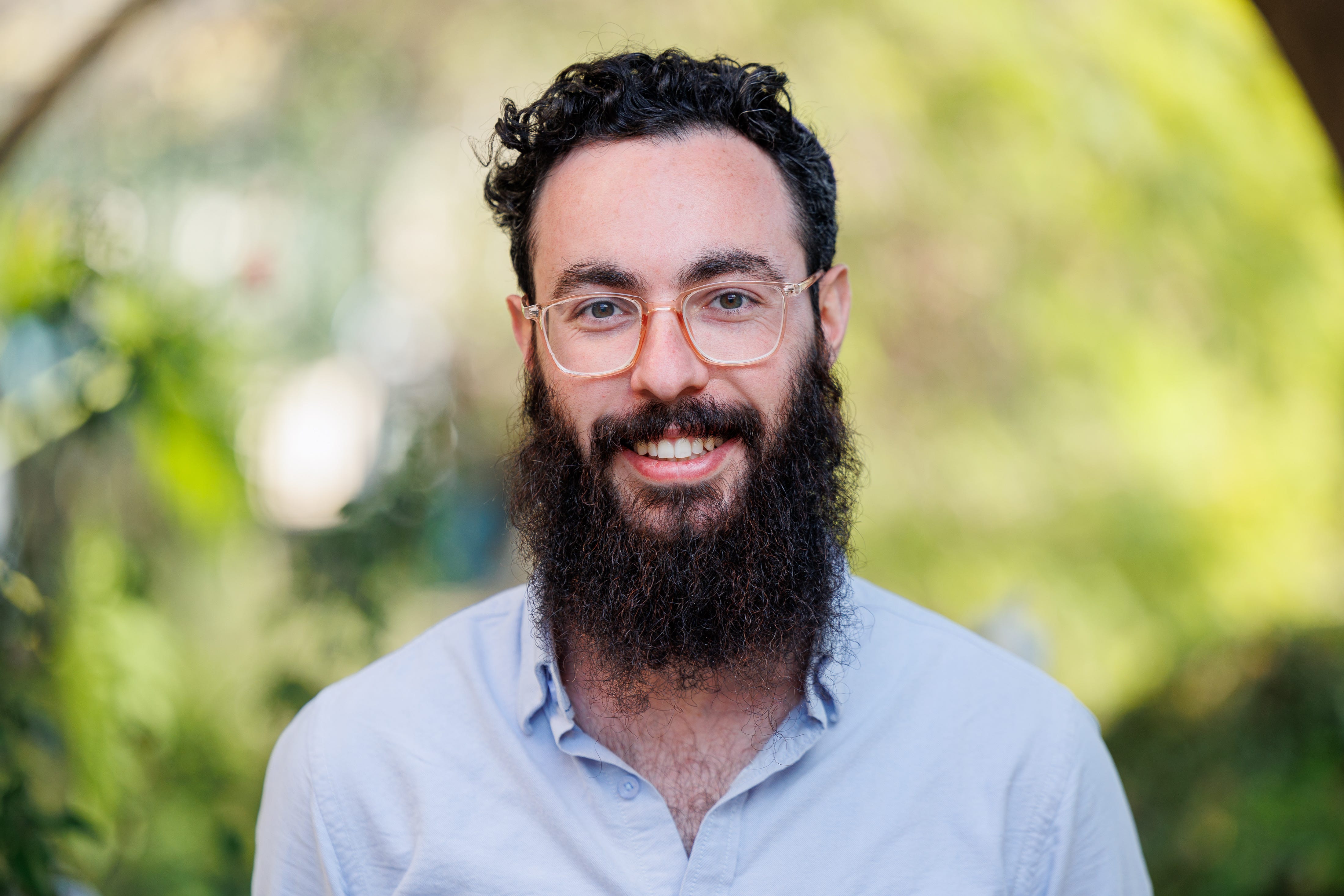This is a photograph of a man who appears to be in his early 30s, centered in the frame, against a blurry, predominantly green background that suggests an outdoor setting with trees and foliage. The man has a pale complexion and is of Arabic or Middle Eastern descent. He sports a very long, curly, dark beard that extends past his shoulders and a thick mustache, both of which partially obscure a broad, warm smile with white teeth. His short, curly black hair shows a slightly receded hairline, and he wears glasses with golden frames. He has thick eyebrows and dark eyes, exuding a happy and approachable demeanor. He is dressed in a light blue, possibly eggshell, button-down work shirt with the top button undone, revealing some chest hair. The photograph's focus and composition draw attention to his facial features and expression, with no other people or text present.